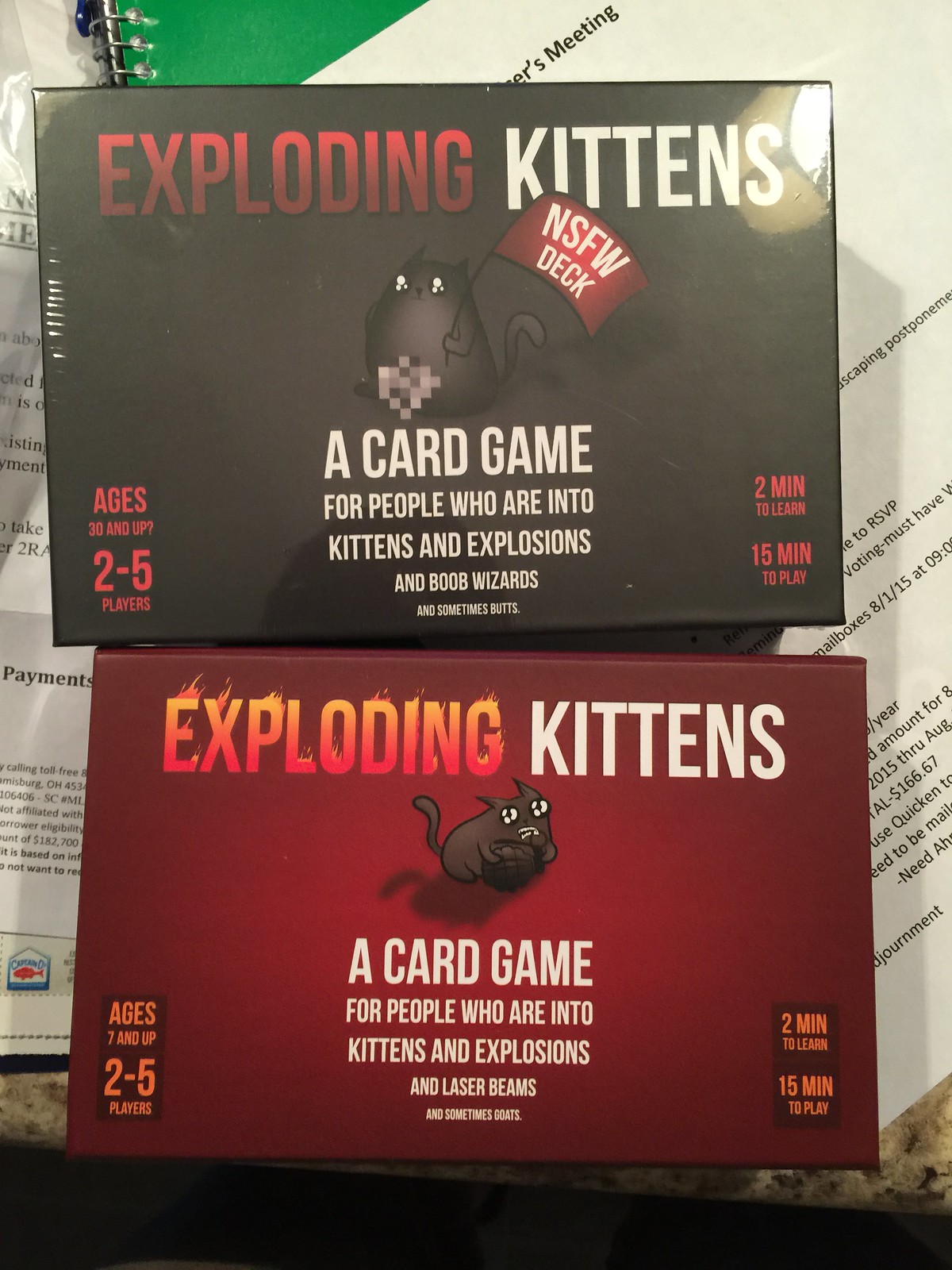This detailed photograph features two boxed card games prominently titled "Exploding Kittens" sitting atop a stack of various pieces of white paper, possibly mail or random paperwork. In the background, the edge of a green notebook is visible. The box on the top is a blackish-gray color, adorned with a picture of a kitten holding a red flag that says "NSFW deck." The description on the box humorously notes it is "a card game for people who are into kittens and explosions and boob wizards and sometimes butts." It also specifies that the game is suitable for ages 30 and up, can be played by 2 to 5 players, and takes only 2 minutes to learn and 15 minutes to play. The box below it is predominantly red, also labeled "Exploding Kittens," featuring a similar kitten illustration. This version is for "people who are into kittens and explosions and laser beams and sometimes goats," marked as appropriate for ages 7 and up. Like the first box, it accommodates 2 to 5 players and requires 2 minutes to learn and 15 minutes to play. Both boxes share eye-catching graphics and witty descriptions, catering to a whimsical and playful audience.